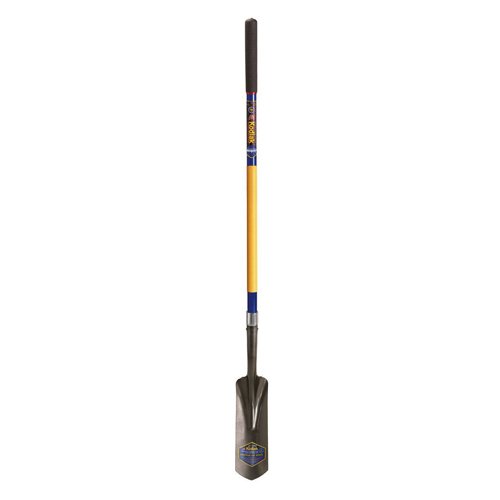This is a high-resolution color photograph of a specialized gardening or digging tool, prominently displayed against a plain white background, likely a stock image. The tool features a long, wooden handle with a black cushioned grip at the top for hand protection. Below this grip is a label with the brand name "Kodiak" printed in yellow. The handle itself is primarily yellow with blue stripes near both ends, adding to its distinctive appearance. The bottom section of the tool is a narrow, metallic shovel that tapers to a pointed tip, and this section is black or dark gray. This shovel appears well-suited for tasks requiring precision, such as trench digging or post hole digging.